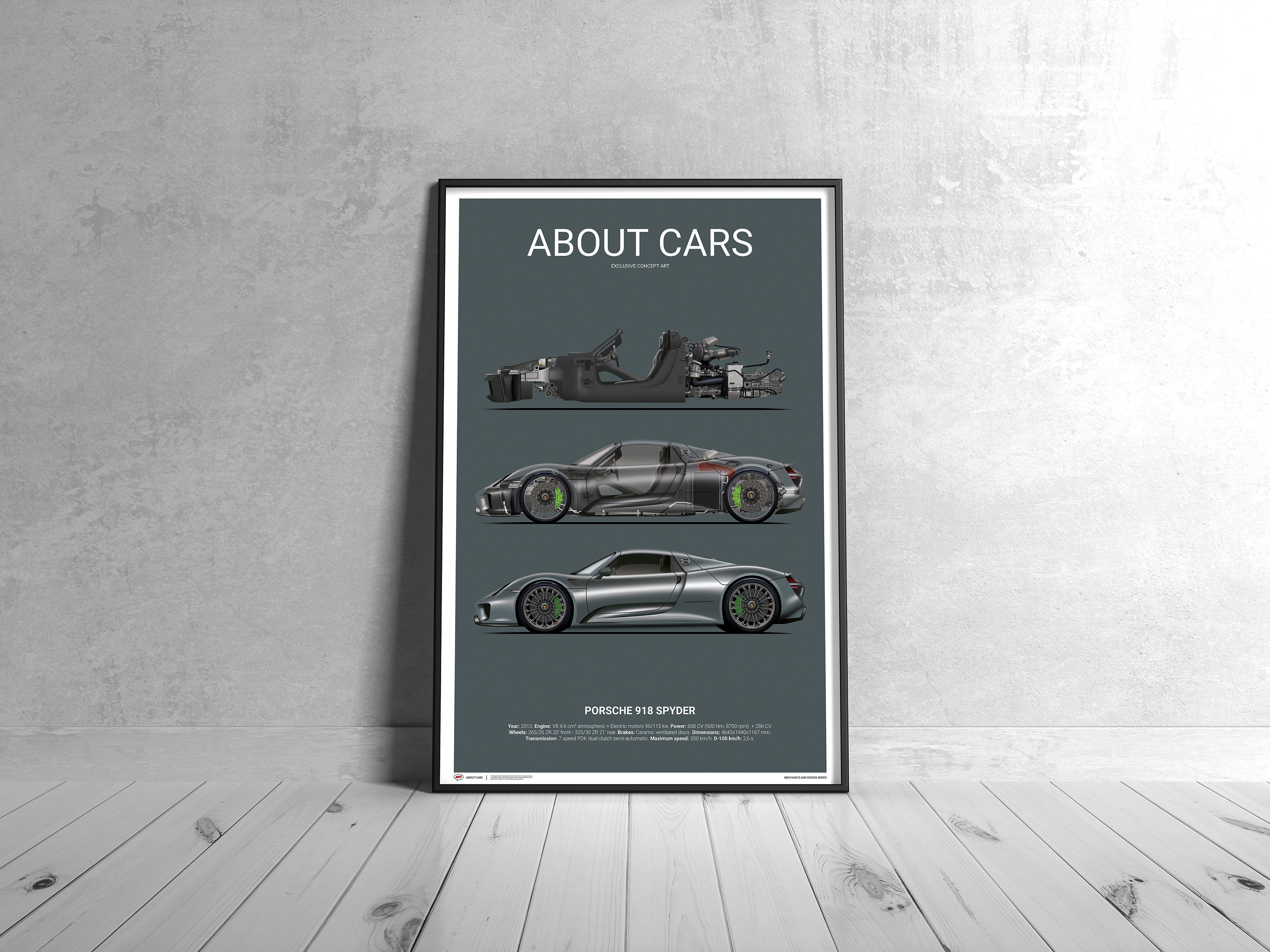This black and white photograph, approximately 5 to 6 inches wide and 4 inches high, captures a minimalist indoor scene. It features a wooden floor with vertical slats that rise about an inch from the bottom edge, topped by a white baseboard. The plain gray wall serves as the backdrop, transitioning from darker tones on the left to almost white on the right. Leaning against this wall, centrally positioned on the floor, is a tall, narrow framed poster. The poster is encased in a simple black frame, which encompasses a white border. At the top center of the poster, bold white text reads "About Cars," with smaller text below stating "Exclusive Concept Art." The main content of the poster is three progressively detailed images of a car. The first image depicts the car in its basic, bare-bones form with a visible interior layout. The second image introduces more structure, incorporating both the tires and additional body outlines. The third and final image showcases the fully completed car. At the bottom of the poster, in white text, it proudly reads "Porsche 918 Spyder." The composition highlights the framed poster as the focal point against the understated elegance of the gray wall and wooden floor.